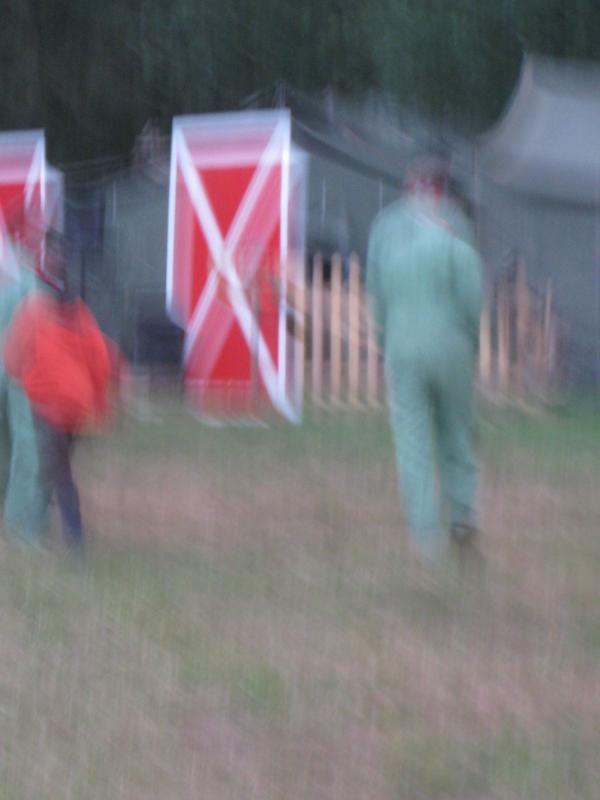In this outdoor scene, a blurred image reveals fragments of a setting characterized by both greenery and patches of dead grass. On the right side, a person dressed in a turquoise jumpsuit and a black hat stands, adding a hint of human activity. To the left, another individual appears in blue jeans paired with a bright orange jacket or hooded sweatshirt, introducing vibrant color contrasts. A wooden picket fence runs along the foreground, providing a rustic touch to the scenery. Dominating the composition is a large rectangular structure that draws the eye—an element resembling a door with a bold white outline, painted in vivid red and prominently marked with a white X.